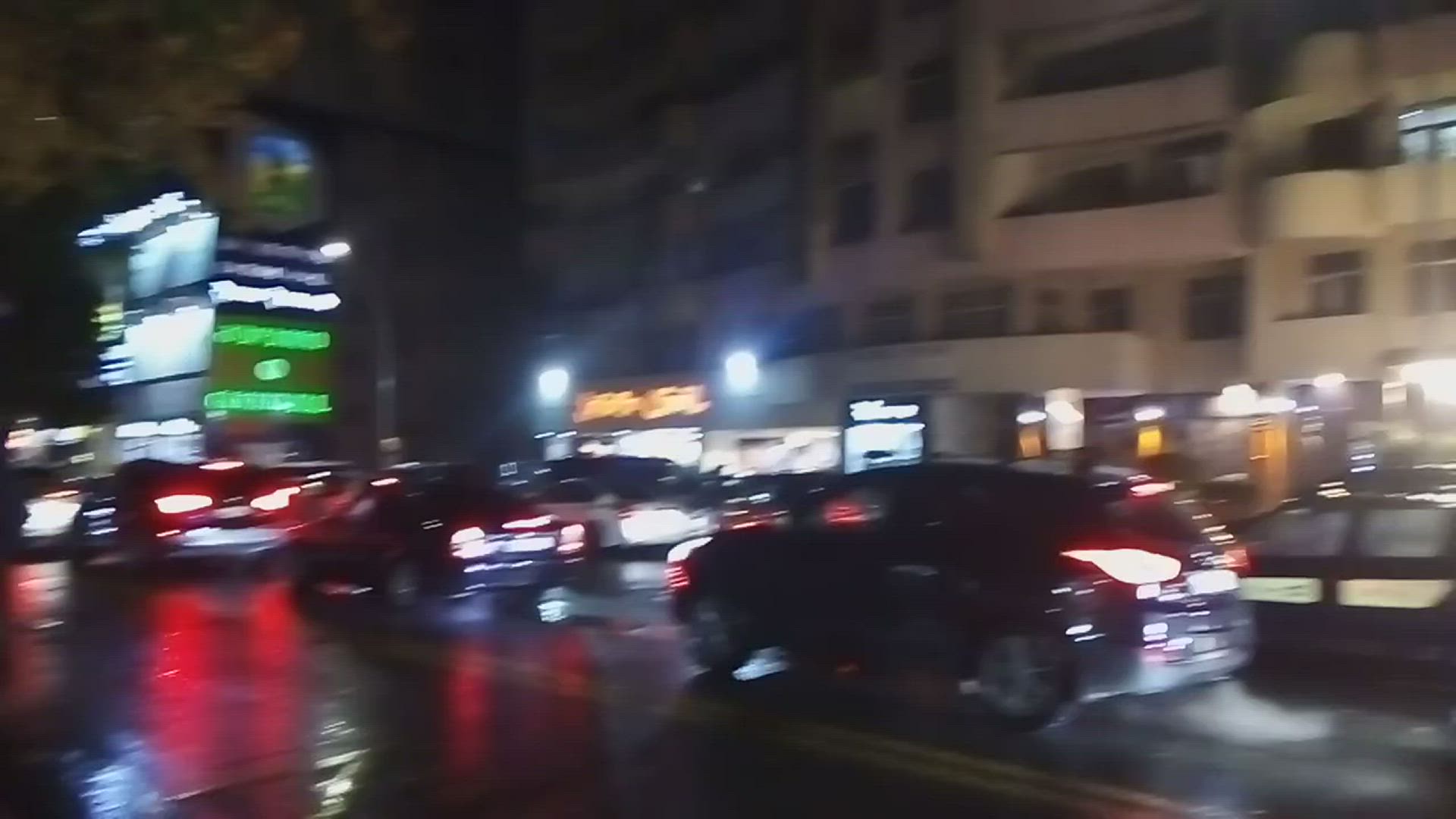This is a nighttime street scene captured in a landscape-oriented photograph with a distinctly busy and rainy ambiance. The road appears wet and shiny, reflecting the lights from numerous cars bustling along the street, primarily traveling from the bottom right to the center left of the image. The photo is quite blurry, adding a sense of motion to the illuminated brake lights and headlights visible among the vehicles. To the right of the image, a large building stands out. Its upper levels are dark, while its lower levels are brightly lit, possibly housing various businesses. Adjacent to this building is a tall, illuminated sign displaying the names of different businesses. Additionally, there's another building further ahead with distinctive green, white, and blue lights. The upper left corner of the scene features the faint outline of a tree, contributing to the photo’s urban-suburban landscape.